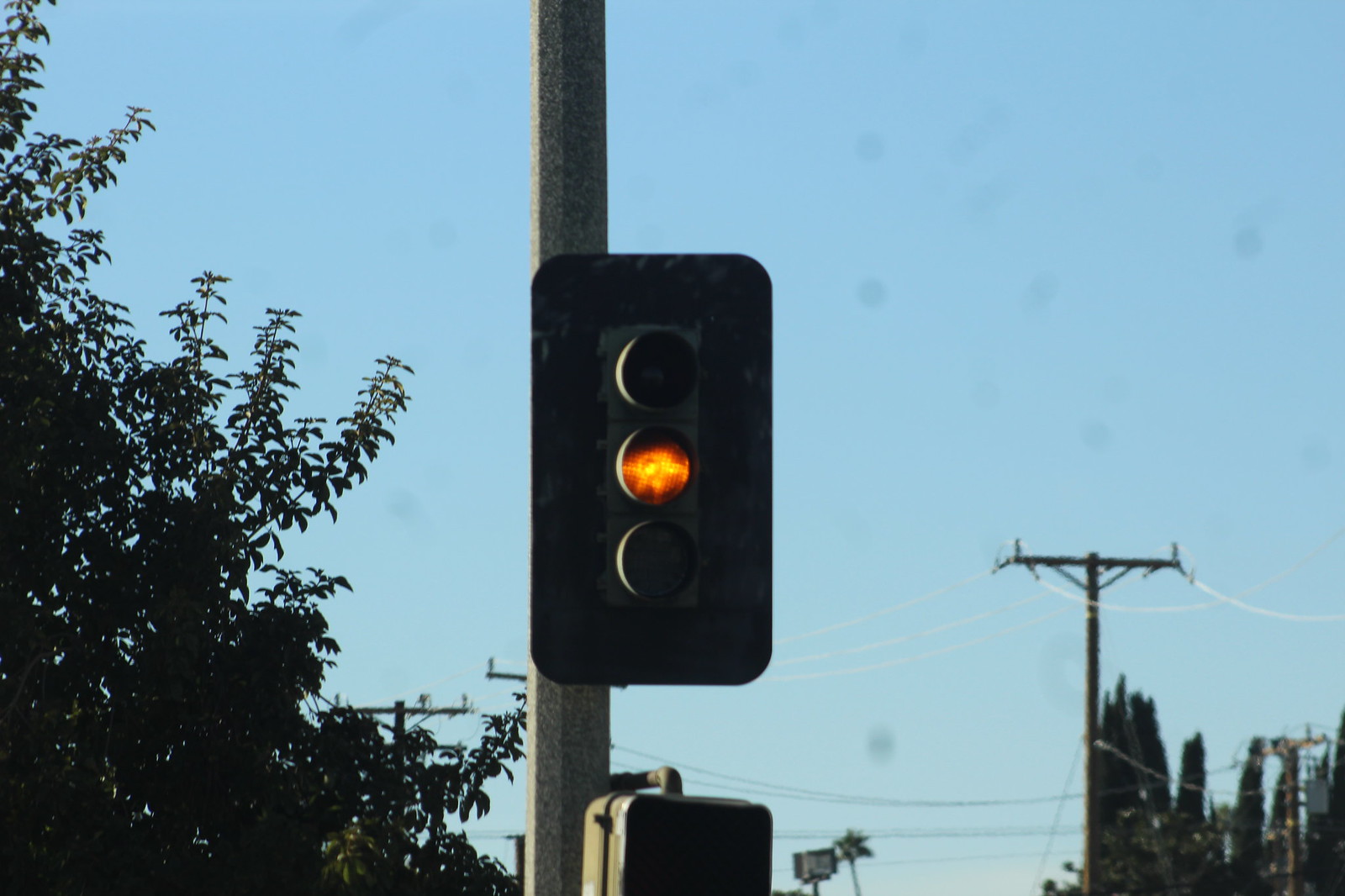The image captures a close-up view of a traffic signal mounted on a silver pole, prominently displaying its yellow light while the other two lights are darkened. The scene is set against a clear, light blue sky, indicating it is a bright and sunny day with no clouds. Surrounding the traffic light, to its left, you can see the top branches and leaves of a tree. Additionally, there are multiple power lines and poles visible in the background on both sides of the traffic light. The overall surroundings, including the trees and power lines, suggest an outdoor setting with an upper, skyward perspective of the terrain. The combination of these elements creates a focused yet detailed view of the traffic signal and its immediate environment.